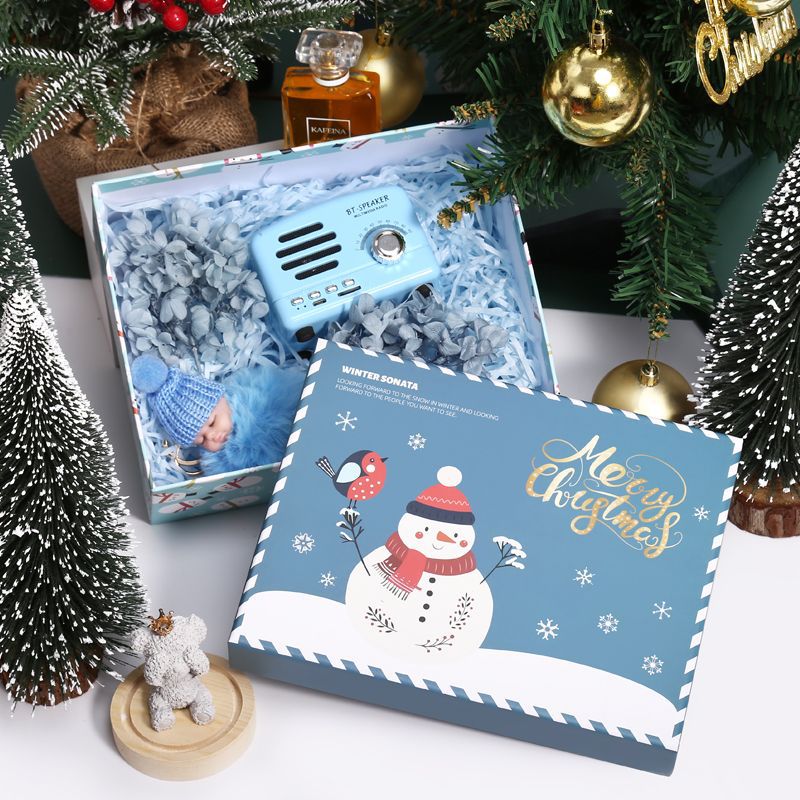The image features an overhead view of a festive, open Christmas gift box set against a white table surrounded by holiday decorations. The box's lid, decorated with a cheerful, cartoonish snowman wearing a red hat and scarf, with a red and black bird perched on its twig arm, displays the message "Merry Christmas" in gold letters. Inside the box, nestled in blue tissue paper, are a small baby blue analog radio labeled "BT Speaker" with silver knobs and buttons, and a realistic baby doll dressed in a blue hat and a fancy blue sweater-blanket combo. Surrounding the box are miniature Christmas trees adorned with white fake snow, bright gold ornaments, cherries, and a brown sack, adding to the holiday scene. A bottle of dark brown cologne with a clear top is also visible among the decorations. Additionally, a small wooden knick-knack featuring a teddy bear with a golden crown, sitting on a wooden piece, adds a charming touch to the display. The bottom half of a large Christmas tree with green pine needles and golden ornaments looms in the background, complementing the festive atmosphere captured in the photograph.